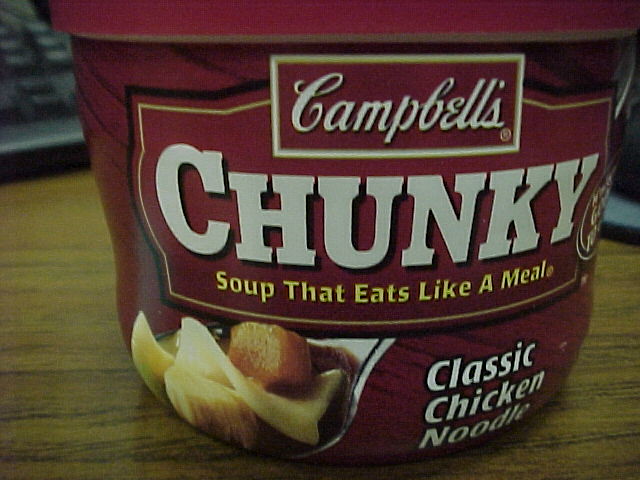On a brown desk, a detailed scene unfolds: in the background, a gray computer keyboard with darker gray keys is visible, and to the right, an assortment of gray and black office equipment is neatly arranged. Dominating the foreground is a large bowl of Campbell's Chunky Soup, still in its original container. The container features a red lid, a bold red label with the iconic Campbell's logo in white, and a white-bordered box filled with red. The prominently displayed "Chunky" text in large white letters is accompanied by the tagline "Soup that Eats Like a Meal" in yellow. At the bottom of the label, "Classic Chicken Noodle" is printed in white letters, alongside a tempting image of a spoonful of soup.